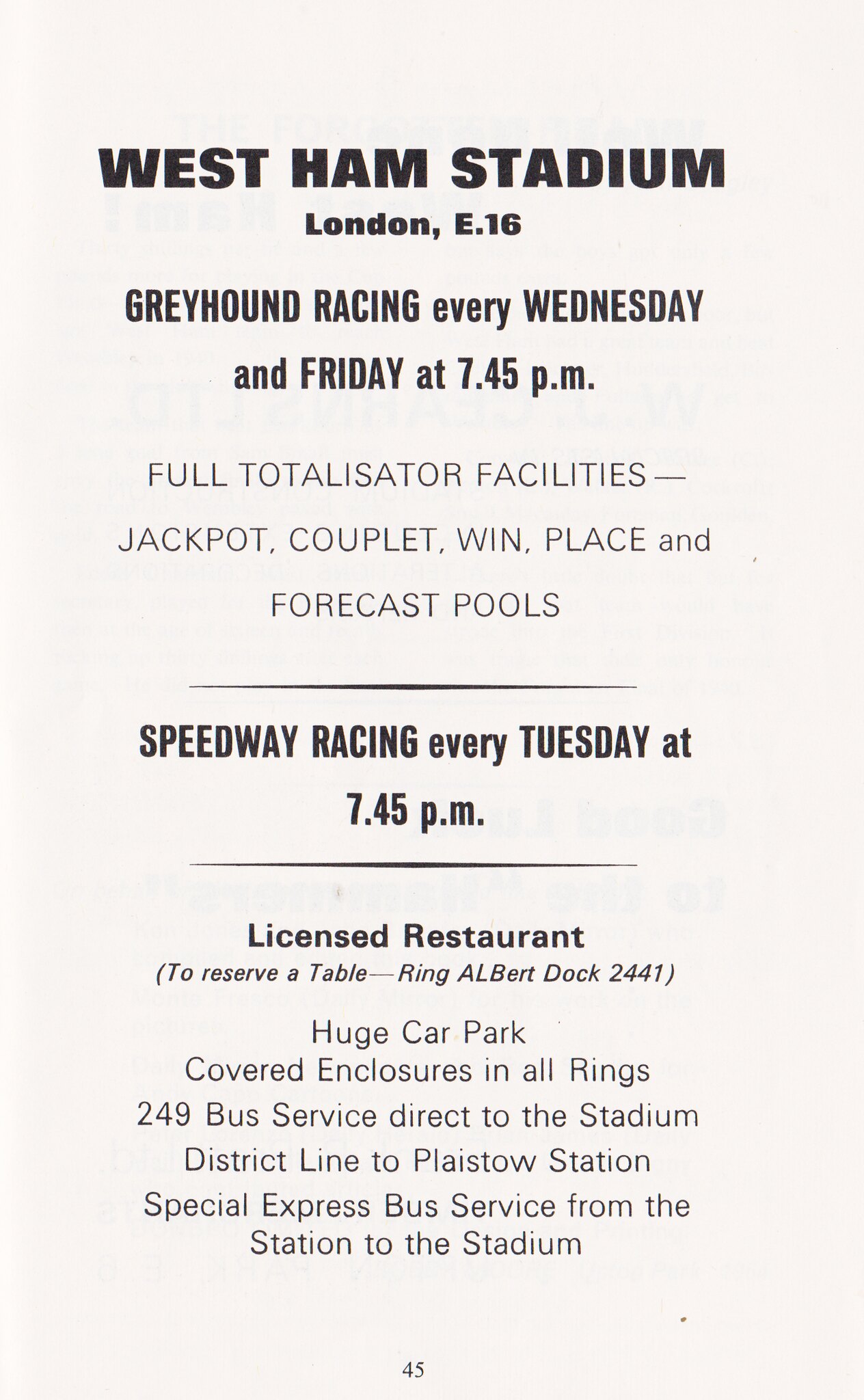This image is a light beige flyer or page promoting events at West Ham Stadium, London E16, prominently featuring black, bold writing at the top that reads "West Ham Stadium, London E16." The flyer advertises Greyhound Racing every Wednesday and Friday at 7.45 p.m., with full totalisator facilities offering jackpot, couplet, win, place, and forecast pools, located towards the center of the page. Additionally, it announces Speedway Racing every Tuesday at 7.45 p.m. It highlights amenities such as a licensed restaurant—reservations can be made by calling Albert Dock 2441—a huge car park, and covered enclosures in all rings. Transportation options include the 249 bus service direct to the stadium, the District Line to Plaistow Station, and a special express bus service from the station to the stadium. The bottom of the flyer displays the number 45, suggesting it may be an excerpt from a booklet or series. The overall design is straightforward with minimal color, primarily black text on a light beige background.